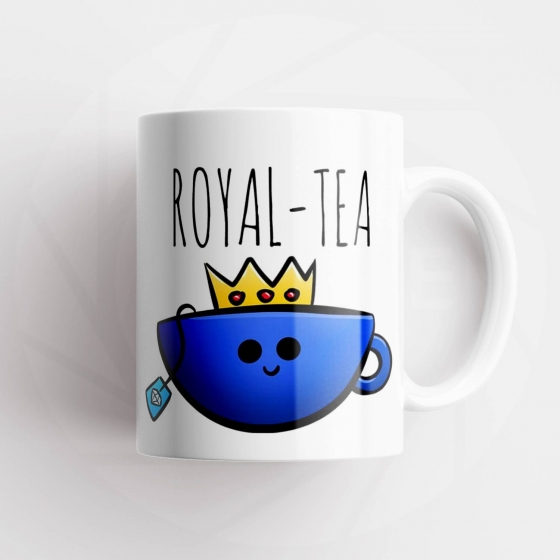The image features a white coffee mug, resting against a plain white background, possibly a table. The mug has a traditional, classic shape with the handle on the right. Prominently displayed at the top in black, all uppercase letters, is the word ROYAL-TEA, cleverly split into two words to create a pun on "royalty." Below this text is a delightful illustration of a blue tea cup with a cheerful face: two black eyes and a smiling, upward curving mouth. The tea cup is adorned with a golden crown featuring three red jewels, emphasizing its regal theme. A tea bag hangs from the left side of the tea cup, its string and blue tag clearly visible. The overall design playfully suggests the notion of "royal tea," marrying the concepts of royalty and a comforting cup of tea.